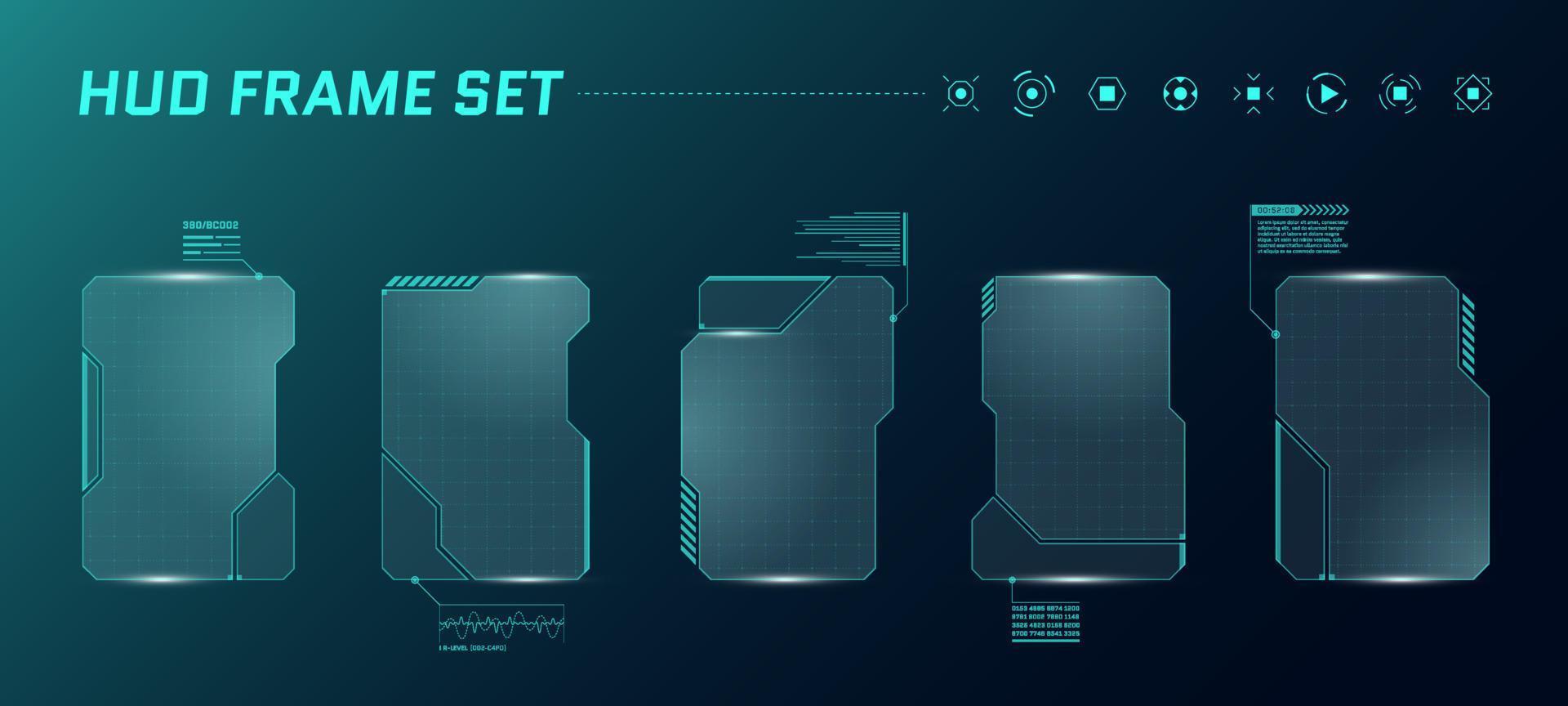This is a detailed, computer-generated image showcasing a HUD (heads-up display) Frame Set, typical in gaming. The image has a predominantly dark greenish-gray to dark green background that transitions to almost black. At the top left, the text "HUD Frame Set" is displayed in bright turquoise. Stretching across the top right are various bright turquoise symbols: two circles, a hexagon with a square center, another circle, a small square with chevron arrows around it, a play button, a stop button with smaller circles and lines, and a square with a diamond and additional chevrons. These symbols serve a decorative purpose within the image.

Beneath the header and symbols, five translucent panels, resembling manila folders, are aligned in a straight row. These panels feature different HUD frame styles, each varying in outline and positioning. Subtle, tiny informational pieces accompany three of the panels, though the text is too small to be legible. The overall layout is straightforward, highlighting the different configurations and designs of the HUD frames, providing a visual representation of their variety and application in gaming environments.